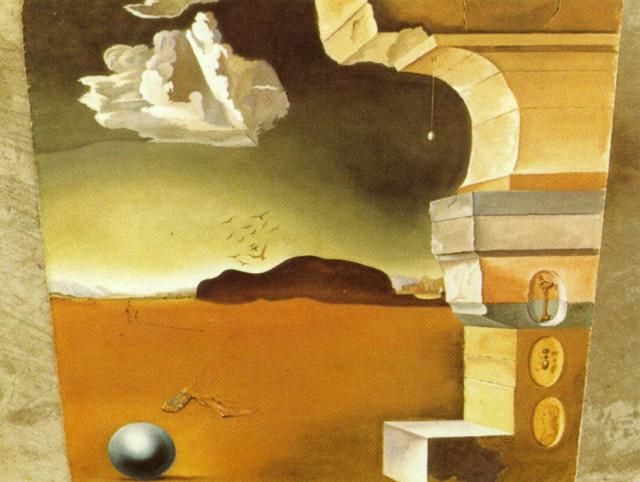The image is a detailed abstract painting with a distinct style reminiscent of Salvador Dali. The artwork features a surreal desert landscape with complex shapes and colors. The background is primarily a dark, overcast sky, with clouds that are lighter along the horizon and a prominent puffy white cloud near the center top. Birds fly above a darker mound or mountain on the horizon, adding to the melancholy of the scene.

The foreground is dominated by an orange, backwards L-shaped structure, which appears to have two button-like elements and a stack of box-like forms in green, orange, and gray on top of it. To the right of this structure is a column-like figure with a mix of tan, white, and beige hues. This column appears sculptural, making use of sloping and curved shapes, echoing the painting's abstract theme.

On the left side of the image, there is a white object resembling a piece of coral, further adding to the surrealism. Below, near the bottom left, a silver sphere with a shadow suggesting a light source from above anchors the composition. This sphere sits on an orange background, contributing to the overall monochromatic palette of whites, beiges, grays, and oranges.

Overall, the painting uses a mixture of geometric and organic forms, accompanied by a subtle but varied color scheme and intricate detailing, creating an evocative and otherworldly work of art.